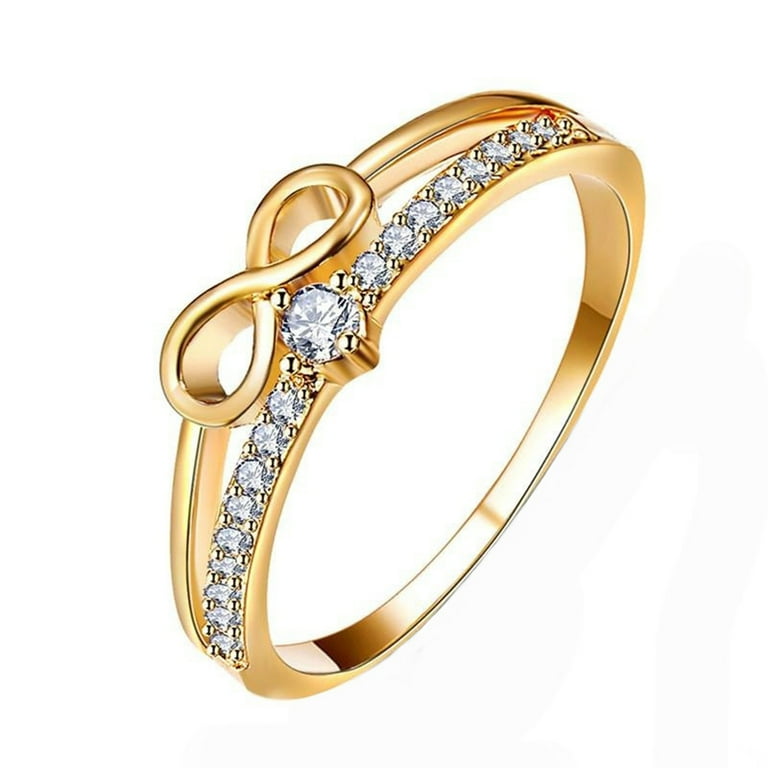The image depicts a stunning, computer-generated gold ring characterized by intricate details and a sense of opulence. The ring features a solid gold band, elegantly polished to a high shine, creating a luxurious appearance. The design of the ring is bifurcated into two distinctive sections. One section showcases a beautifully molded infinity symbol, which is seamlessly integrated into the structure of the ring, also rendered in gold. The second section is adorned with numerous small, equally spaced diamonds that extend from one side to the other, reflecting light brilliantly. 

Central to the ring’s design is a larger, prominent diamond, bordered by four golden pearls at each corner, adding to its grandeur. This central diamond is noticeably bigger than the rest and is securely embedded within the golden frame. The attention to detail is evident in how the smaller diamonds are meticulously inlaid along the top edge of the band, avoiding any engravings or marks, thus maintaining a sleek and pristine look.

The ring appears to float in an empty, white background, emphasizing its aesthetic features. The lack of any additional background elements allows the viewer to appreciate the craftsmanship and the reflective gold surface of the ring. Overall, this gold ring, with its infinity symbol and array of diamonds, exudes a sense of elegance and high value, making it a piece of exquisite jewelry.